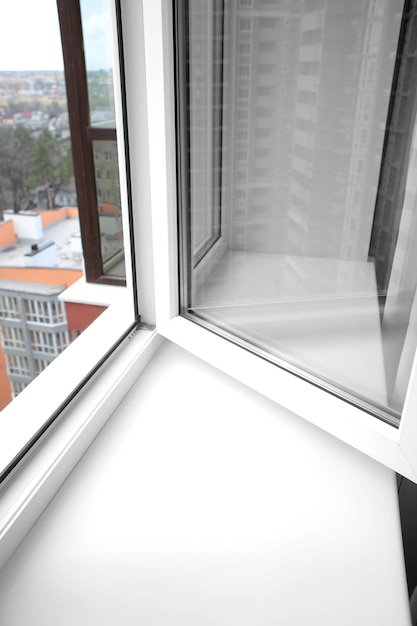The image is a photograph taken from the perspective of an open window, revealing an urban cityscape. The window, positioned to the left and open inward, dominates the foreground. The windowsill, wide and white, extends about 70% across the bottom of the frame, leading to the interior of a mostly white room, possibly an office. Reflections of nearby buildings are visible in the glass of the open window. Outside, a city environment unfolds with a mix of concrete skyscrapers, apartment buildings, and treetops. The nearest building, tinged with pinkish, reddish, and tannish hues, adds a splash of color against the otherwise predominantly white and subdued tone of the scene. In the distance, numerous high-rises and balconies form a skyline under a cloudy sky.